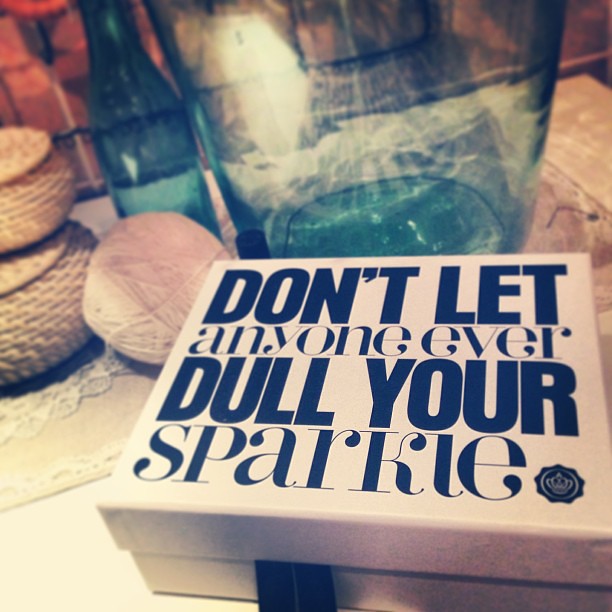This photograph, taken indoors in a dimly lit room during daytime, features several objects arranged on a wooden desk. Dominating the bottom right corner is a white square box with a brownish tinge. The lid of the box, designed to lift off without folding, prominently displays the motto "Don't let anyone ever dull your sparkle" in artistic black serif font, with "don't let" and "dull your" emphasized in bold, condensed letters. To the left of the box, near the center and stretching upward towards the top left corner, are two woven wicker baskets stacked one on top of the other, accompanied by a ball of white yarn. Adjacent to these, towards the top left, there are a couple of bottles. In the upper right corner of the image, a light blue-tinted glass jar can be seen. The scene evokes a sense of eclectic organization, perhaps suggesting an antique room with a mix of various items in white, tan, black, green, red, and brown hues.